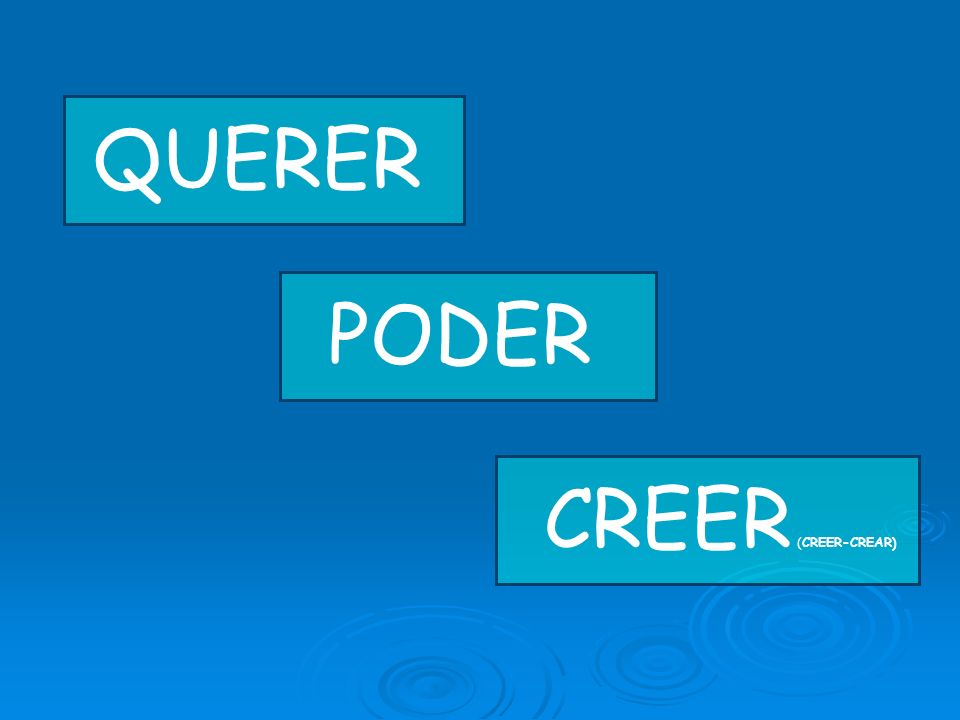The image appears to be a PowerPoint slide with a gradient background transitioning from cerulean at the top to a lighter blue-jean hue at the bottom, adorned with subtle water ripple effects along the bottom right. Positioned diagonally from the top left to the bottom right of the slide are three teal text boxes. The top left box contains the word "QUERER" in white font, the central box holds "PODER," and the bottom right box displays "CREER," which is also accompanied by the parenthetical "CREER - CREAR" in small white lettering. The overall aesthetic is minimalistic yet visually engaging, with the water-like ripples adding a dynamic touch to the serene blue backdrop.